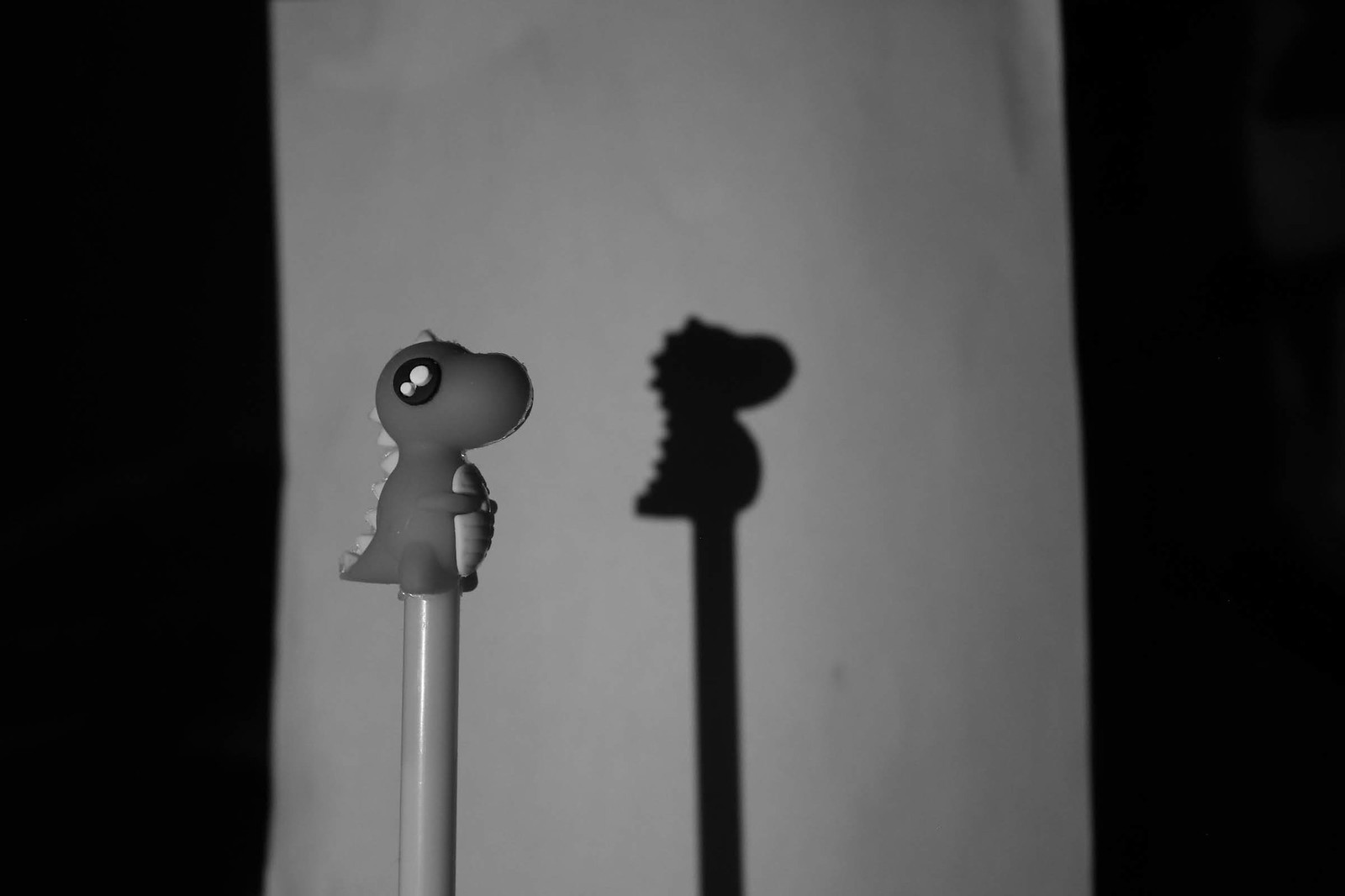The image is a black-and-white artistic photograph taken indoors, presenting a small toy figurine perched atop a metal rod or stick. The figurine resembles either a dragon or dinosaur, characterized by scales running along its spine, a large, bulging belly, and prominent, round eyes. The creature is facing to the right, with its little arms resting on its lighter-colored belly. The background features a white or light-colored tapestry that displays the figurine's shadow, adding to the artistic composition. The surrounding scene is enveloped in darkness, with the lighted backdrop framed by darker bands or shadows, creating a dramatic and focused spotlight effect on the toy and its shadow.